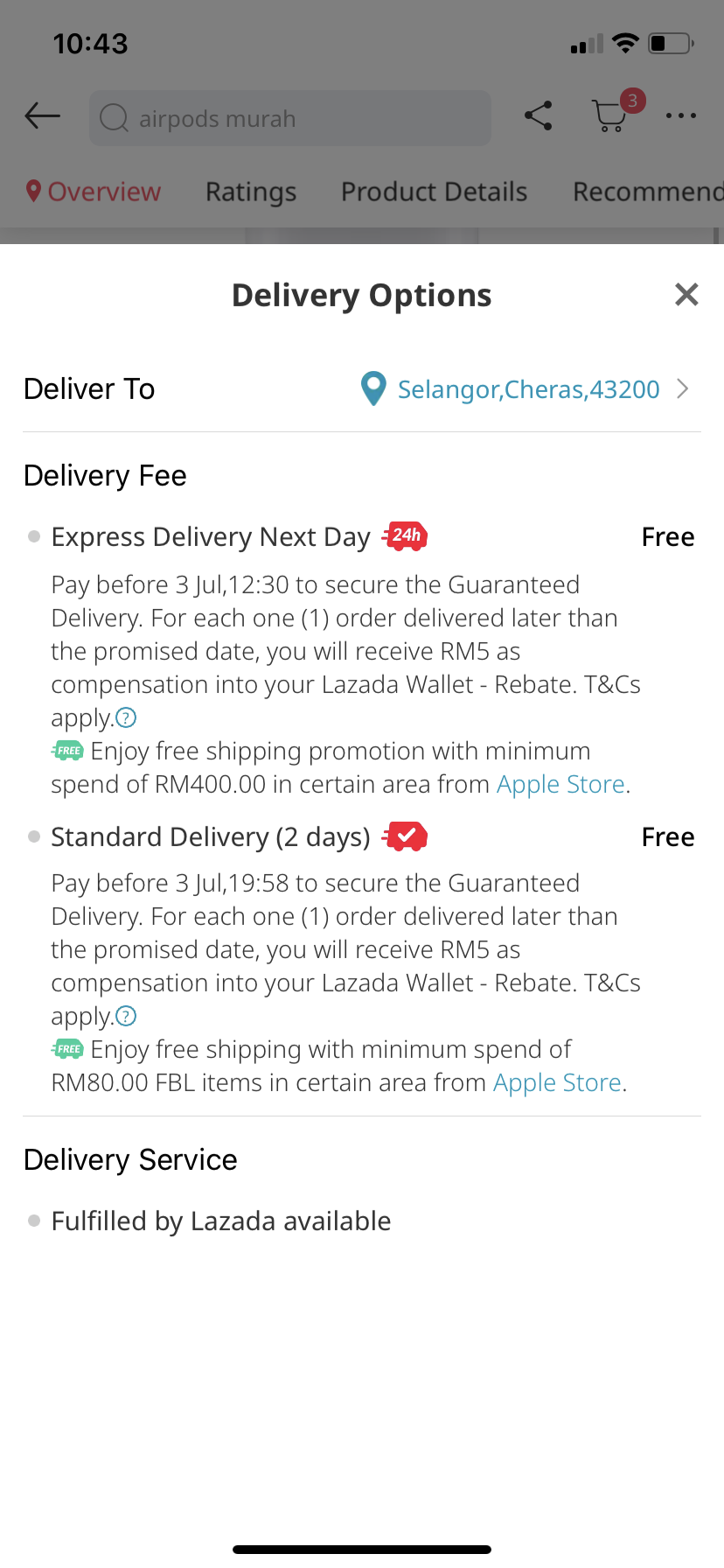**Caption:**

This screenshot captures a pop-up within a mobile application, displaying various delivery options. The pop-up is set against a white background and extends approximately three-quarters up the screen. 

At the top center, the header features the bold black text "Delivery Options." On the top right, there is a dark gray "X" for closing the pop-up. Towards the left of the header, the text "Deliver to" is displayed in black. In the bottom right corner of the header, a teal blue map pin icon is followed by the blue text "Selangor, Charas, 43200," accompanied by a gray right-pointing arrow. A thin, light gray separating line runs beneath the header.

The body of the pop-up starts with "Delivery Fee" in black text at the top left. Below this, there are two sections of information, each preceded by light gray bullet points. Each section contains black headline text followed by light gray descriptive text. Towards the far right side of these sections, "Free" is prominently displayed in black.

1. **Express Delivery (Next Day):** 
   - Icon: A pink van with white "24H".
   - Details: "Pay before 3 July 12:30 to secure the guaranteed delivery. For each order delivered later than the promised date, you will receive RM5 as compensation into your Lozada wallet - rebate. T&Cs apply."
   - Additional Info: A bright blue question mark icon encircled in blue is present to the right.

2. **Standard Delivery (Two Days):**
   - Icon: A green van with white "Free".
   - Details: "Enjoy free shipping promotion with a minimum spend of RM400.00 in certain area from Apple Store."

These comprehensive details guide the user on the available delivery options and respective conditions.